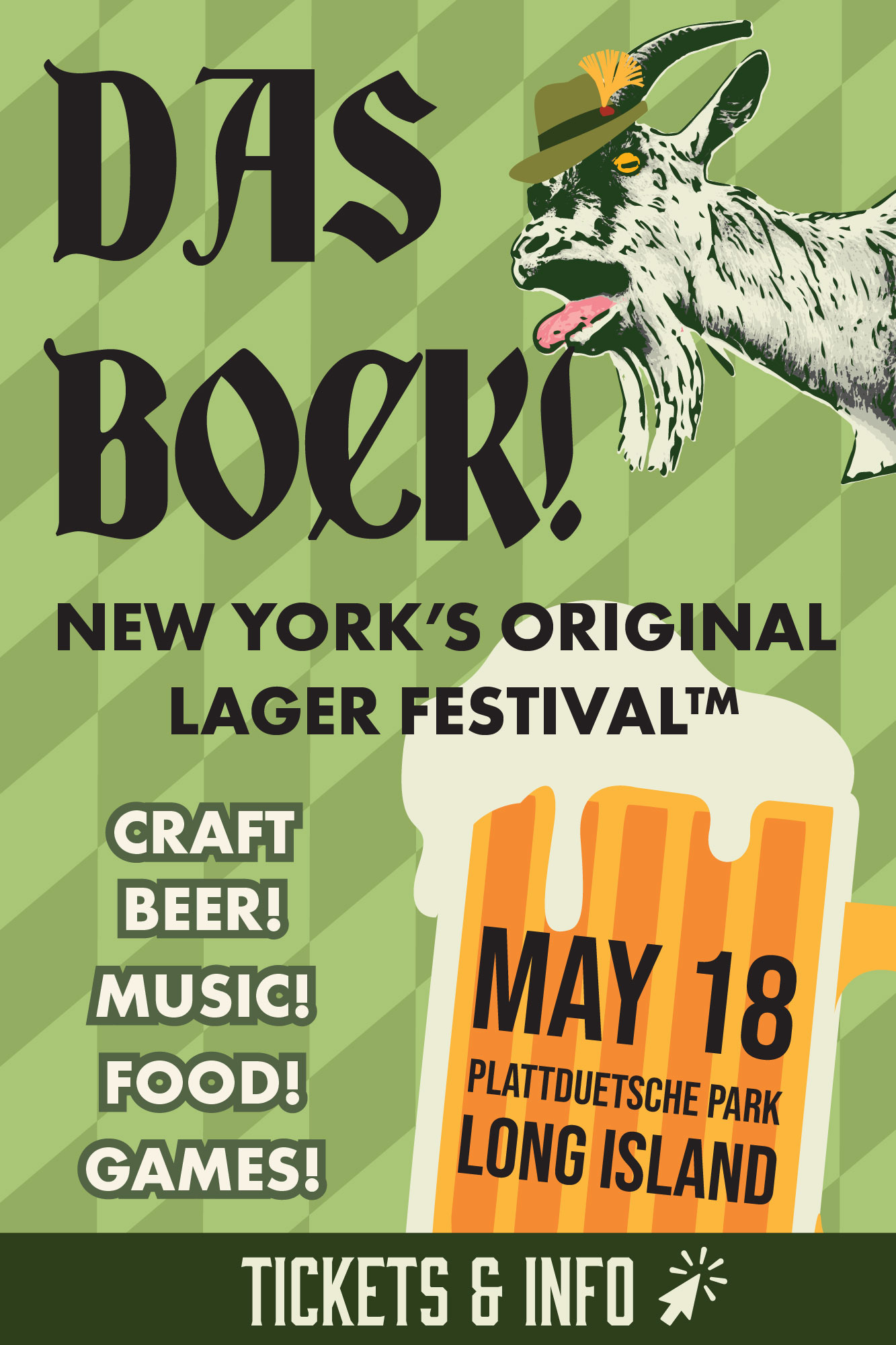The festival poster features a captivating design in shades of light green to dark green, with highlights in yellow and orange. At the top, in prominent dark Old English style lettering, it announces "Das Bock!" with an exclamation point. Below this, in smaller black text, the poster identifies the event as "New York's Original Lager Festival." The left-hand side lists attractions like "Craft beer, music, food, and games" in white lettering with a green outline. On the right, in black letters on an overflowing beer stein graphic outlined in white with yellow and orange accents, it provides the details: "May 18th, Plattdeutsche Park, Long Island." 

A quirky white goat, with its tongue sticking out and a green German hat perched atop its head, adds a whimsical touch to the visual. The background is decorated with alternating diamond patterns in light and medium green, enhancing the festive vibe of the poster. At the bottom, an olive green banner marked "Tickets and info" features an arrow, suggesting interactivity, like pressing a button.